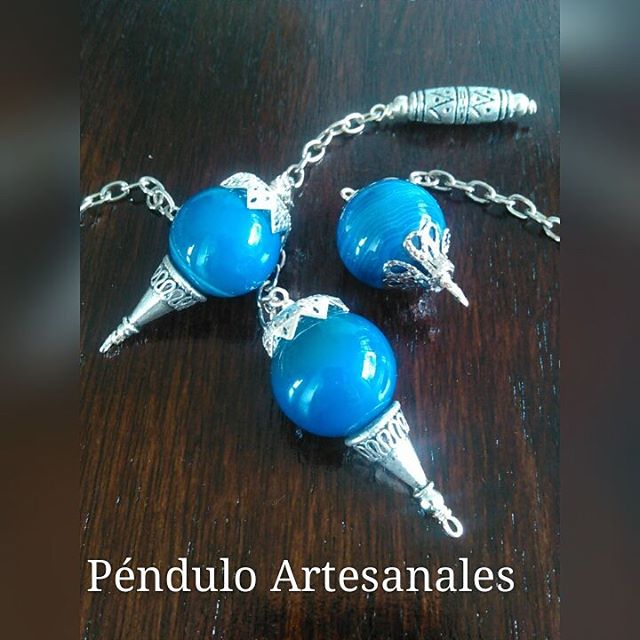Three artisanal pendants are displayed on a dark wooden table with a rich wood grain. Each pendant is crafted from a sky-blue globe, reminiscent of pearls but with a bright blue hue. The globes are capped with silver tops, resembling the metal tops found on Christmas ornaments. These caps are connected to short silver chains, which in turn are attached to intricately engraved silver handles. The bottom of each globe is adorned with a decorative point, evoking the look of a plumb bob used by land surveyors. White text at the bottom of the image reads "Pendulo Artesanales" in Spanish.